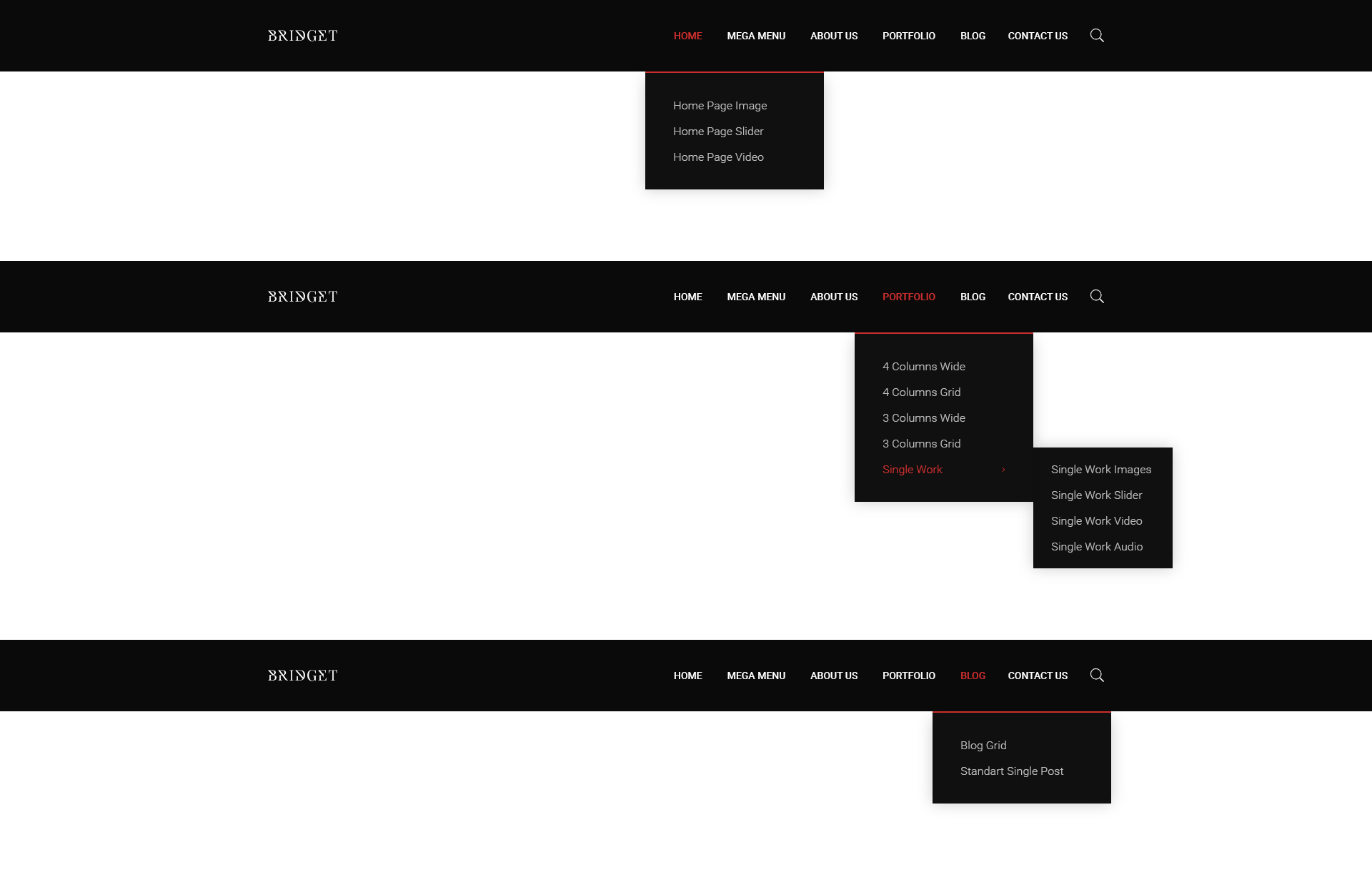The screenshot captures the top navigation bar of a website, showcasing various dropdown categories. On the far left, a tab labeled "Budget" is prominently displayed. Moving to the right, the navigation menu includes several tabs: "Home," a partially obscured tab that appears to start with 'Mega,' likely "Mega Menu," followed by other blurred-out tabs. The second-to-last tab reads "Blog," while the final tab says "Contact Us."

Upon hovering over "Home," a dropdown menu is revealed, listing subcategories such as "Home Page Image," "Home Page Slider," and "Home Page Video." In the center of the navigation bar, the "Portfolio" tab unveils further options including "Four Columns Wide," "Four Columns Grid," "Three Columns Wide," "Three Columns Grid," and "Single Work."

Similarly, hovering over "Blog" exposes additional categories: "Blog Grid," and something resembling "Star," possibly indicating a featured section or format, alongside a "Single Post" option. The entire menu's text appears somewhat blurred, but the general structure and organization of the navigation elements are discernible.